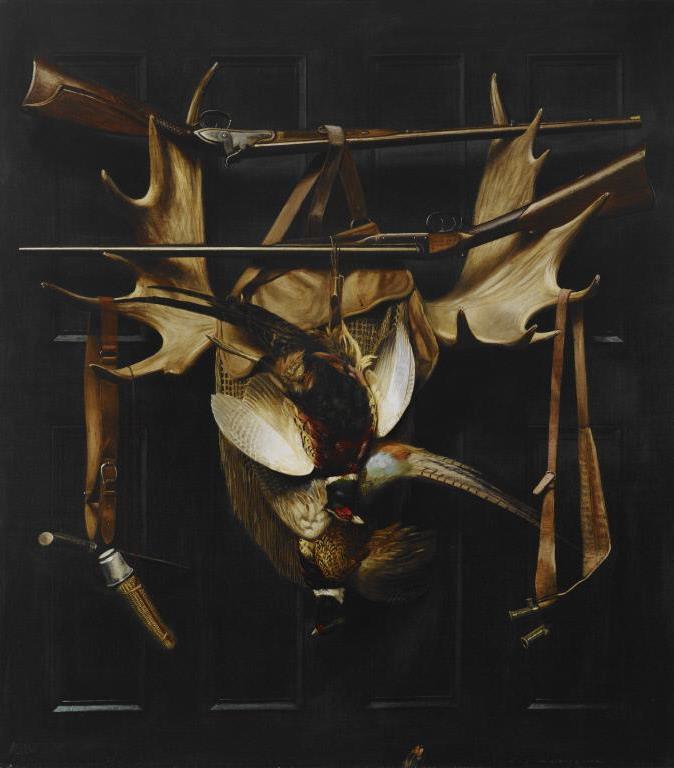The image is a highly detailed digital painting, employing the trompe l'oeil technique to create a realistic illusion. The backdrop features a dark, black door or wall with two rows of rectangular indents, four across and two down. In the center, prominently displayed, is a pair of moose antlers. Balanced horizontally on top of the moose antlers are two rifles, both positioned upside down. The rifle at the top has its stock on the left and barrel on the right, while the rifle below has its stock on the right and barrel on the left. From the barrel of the top rifle hangs a brown bag attached via straps, and two pheasants dangle upside down by their feet from the center of the lower rifle. Additional straps are hanging from the second last point on the left side and the third last point on the right side of the antlers, though the contents they hold are unclear. The painting uses a variety of brown tones, and a sheen on the gun barrels and highlights on the bird's feathers contribute to its lifelike appearance.